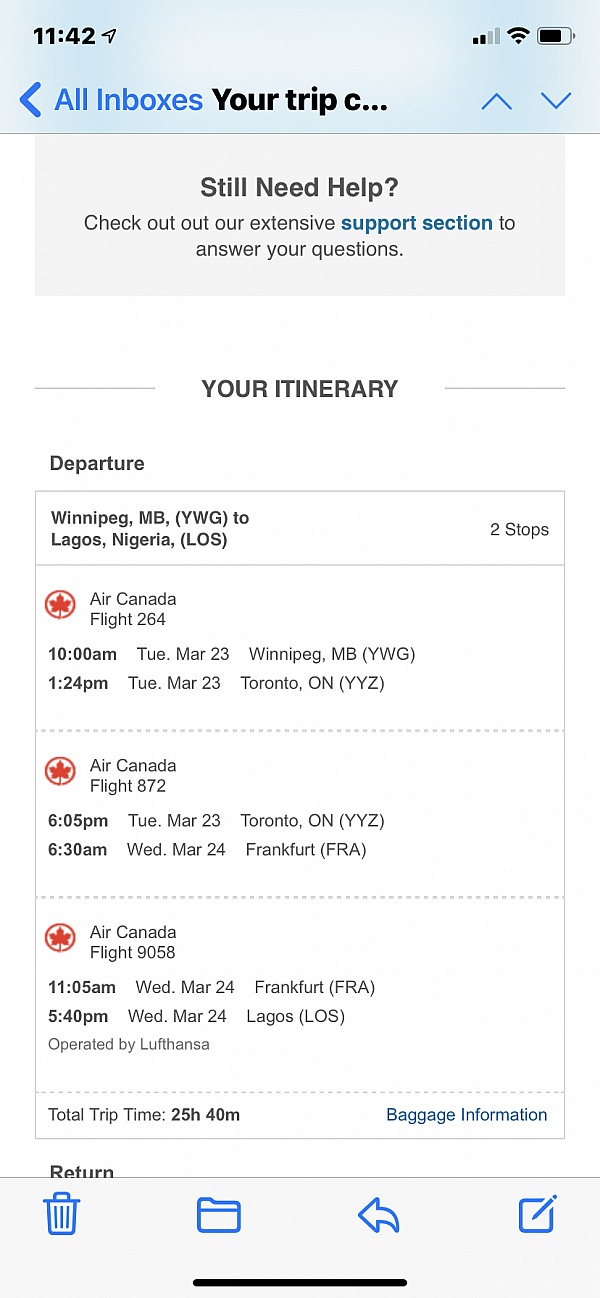This image is a detailed screenshot of an iPhone mail app displaying an email containing a flight itinerary. The email reveals a complex travel route from Canada to Nigeria, departing from Winnipeg (YWG) and arriving in Lagos (LOS) with two layovers. The journey includes stops in Toronto and Frankfurt, accumulating to a total travel time of 25 hours and 40 minutes. The device interface is distinctly iOS, featuring the traditional elements such as the time displayed in the upper left corner (11:42), battery life indicator, and blue-colored icons and text boxes. At the bottom of the screen, there are navigational icons for trash, folder, reply, and composing a new email.